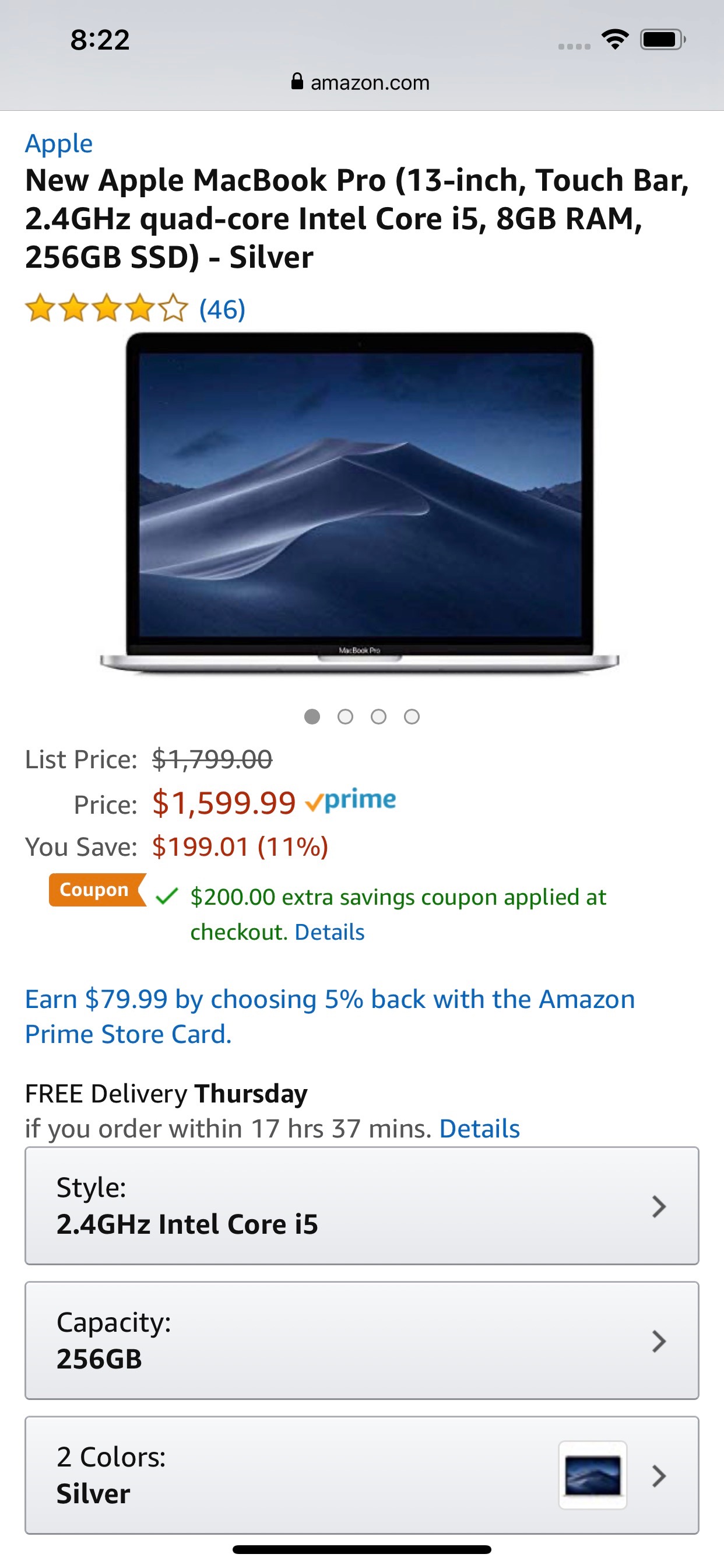The image displays a screenshot of a smartphone showing an Amazon product page. At the top, a gray banner includes a timestamp "8:22" in the center, followed by a lock icon and "amazon.com." To the right are four small square icons, a full Wi-Fi signal icon, and a nearly full battery icon.

The product featured is the Apple MacBook Pro 13-inch with a Touch Bar, powered by a 2.4 GHz quad-core Intel Core i5 processor. It has 8 GB of RAM and a 256 GB SSD, and the model showcased is in silver. This laptop has received an average rating of 4 out of 5 stars based on 46 reviews. The listed price is $1,799, but with Amazon Prime, it is available for $1,599, offering a savings of $199.01, which is an 11% discount. Additionally, there is a coupon for an extra $20 savings applied at checkout. A "Details" link follows the coupon information.

Beneath this, there is a note that customers can earn $79.99 back by choosing 5% back with the Amazon Prime Store Card. The delivery information states that free capped-out delivery is available by Thursday if the order is placed within 17 hours and 37 minutes, with another "Details" link below.

Further down, three gray boxes with right-facing arrows provide additional options:
- Style: 2.4 GHz Intel Core i5
- Capacity: 256 GB
- Color: Silver